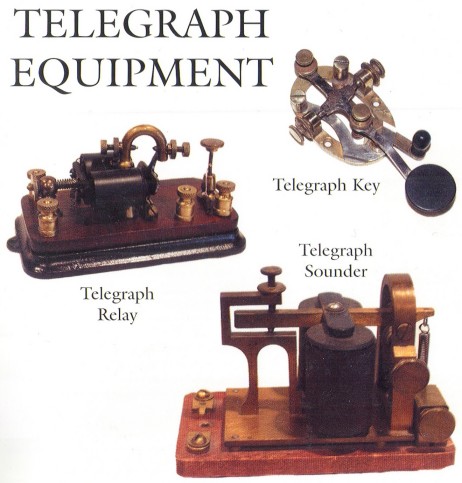The photograph is a detailed, full-color combination print of historical telegraph equipment, set against a simple white computer screen background. The image is square with no borders, dominated by the title "TELEGRAPH EQUIPMENT" in bold, all-capital black letters at the upper left corner. The photograph showcases three distinct components of telegraph machinery, each clearly labeled in black text beneath their respective images.

On the left is the "TELEGRAPH RELAY," depicted as a vertical assembly with several cylindrical objects mounted on a wooden base, featuring a combination of darker wood and brass elements. To the upper right, the "TELEGRAPH KEY" is presented, characterized by a metal ovular shape with a prominent black plastic circle attached to a stainless steel rod. Finally, at the bottom, the "TELEGRAPH SOUNDER" is displayed on a wooden pedestal, incorporating both metal and black plastic parts. The overall aesthetic of these devices suggests they date back to the 1800s, giving a nostalgic glimpse into early telegraphic communication technology.